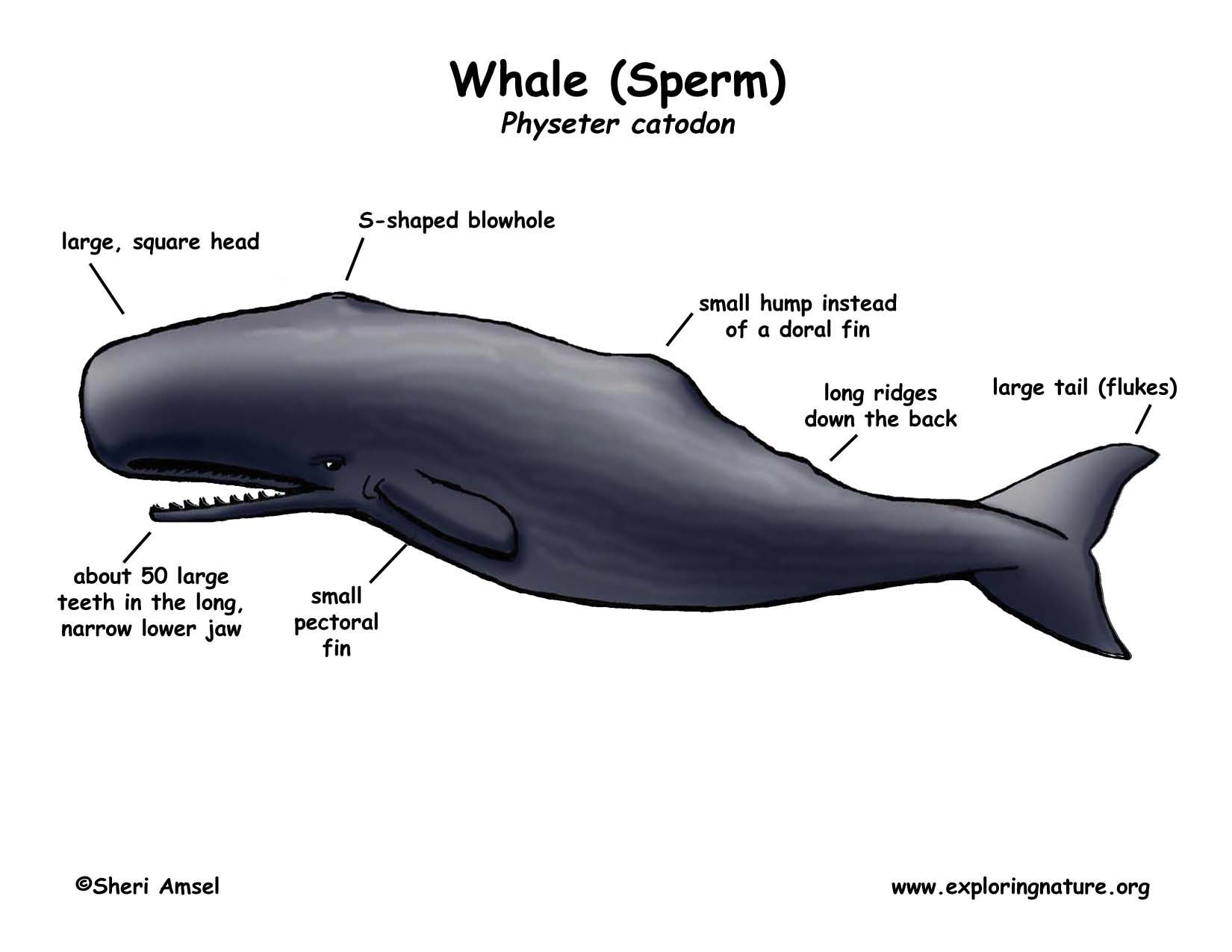This detailed infographic depicts a sperm whale with various anatomical features labeled, suggesting an educational purpose. At the top of the image, the text "Whale (Sperm)” is prominently displayed, followed by the scientific name "Physeter catodon," which is spelled out as "C-A-T-O-D-O-N." The centerpiece of the graphic is an outlined whale, colored in shades of gray with wavy white lines, positioned leftwards with its mouth open to the left side of the screen, exposing around 50 large teeth in its long, narrow lower jaw. Surrounding the whale are labels indicating its body parts: a "large square head" with a line pointing to its head, an "S-shaped blowhole" at the top, a "small hump instead of a dorsal fin" towards the middle, "long ridges down the back," and a "large tail (flukes)" at the right end. Additionally, the whale has a "small pectoral fin" indicated on the underside. The graphic utilizes a comic sans font for all text, reinforcing its illustrative and instructive nature, with the URL "www.exploringnature.org" and the name "Sherry Amsel" noted at the bottom. The overall use of white, black, and various shades of gray enhances the diagram's clarity and visual appeal.